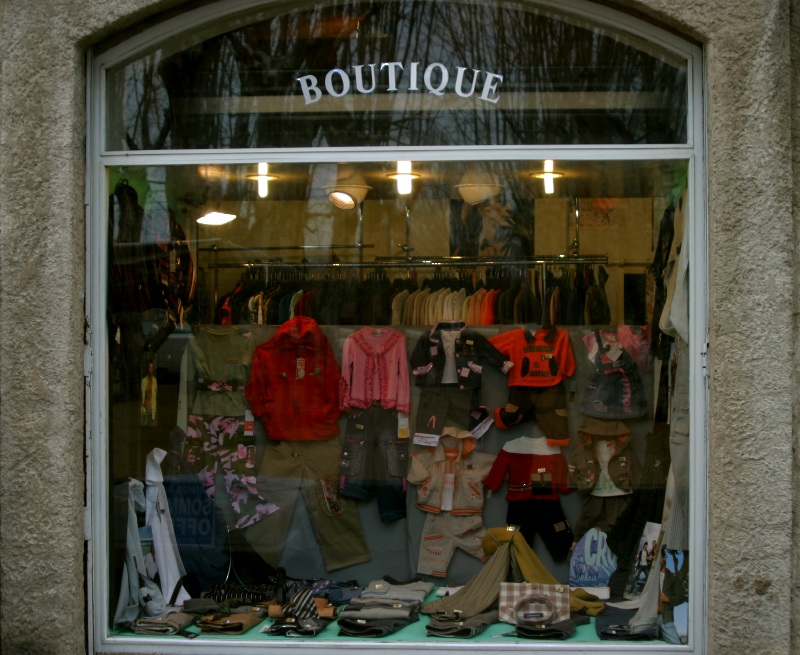This image depicts the exterior of a boutique clothing store. The storefront is framed by gray brick and features a large window with "boutique" prominently displayed at the top. Through the window, various men’s, women’s, and children's garments are visible, including dresses, shirts, pants, and shoes. Notably, the clothing displays contain a mix of early 2000s and late 90s styles, with an array of colors dominated by pink, black, and hints of red. The boutique's interior showcases a well-lit space with fancy lighting and a somewhat cluttered yet diverse collection of outfits. Above the front display, there is a sizable rack filled with clothes on hangers, offering a glimpse of the rich assortment available inside the store.